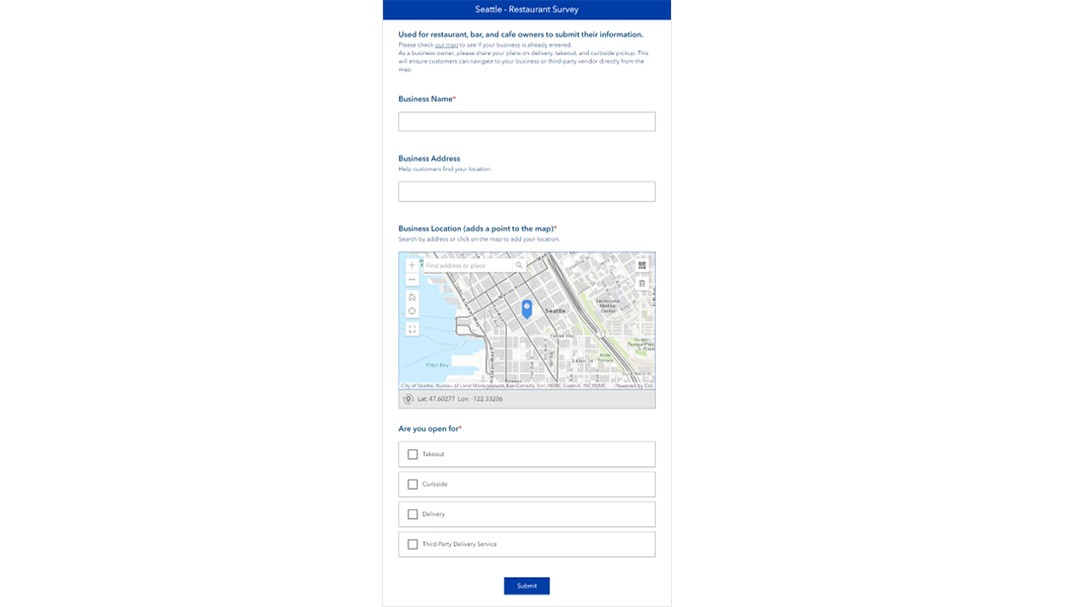The image depicts a page featuring a detailed map aimed at restaurant, bar, and cafe owners in Seattle. At the top, a heading reads "Seattle Restaurant Survey." The purpose of the survey is to gather information from business owners about their establishments. The page urges owners to check the map to see if their business is already listed and to update their information if needed. Business owners are encouraged to share their plans regarding delivery, takeout, and curbside services to enable customers to navigate directly to their business or a third-party vendor via the map. Essential details such as the business name, address, and exact location on the map can be added by searching the address or clicking on the map. The survey also collects information on whether the business is open for takeout, curbside pickup, delivery, or uses third-party delivery services.